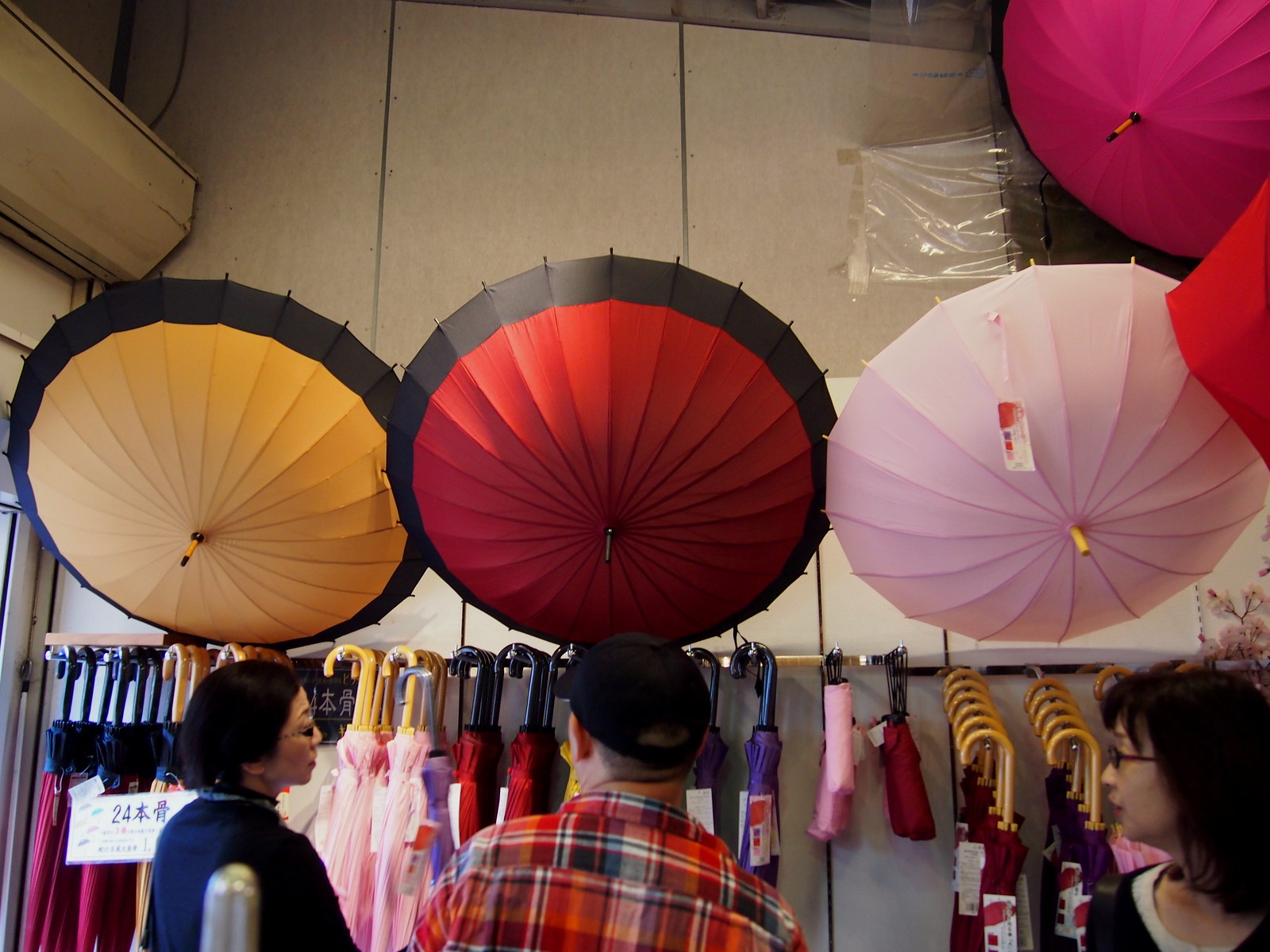In the image, three people are shopping for umbrellas in a brightly lit store. The two female-presenting individuals, who have short dark hair and glasses, and the male-presenting individual, who is wearing a black ball cap and a red plaid shirt, all face away from the camera, with the women's side profiles visible. The women are both dressed in dark shirts, with the one on the left possibly wearing a jacket.

They are browsing a vibrant display of umbrellas, predominantly featuring hues of pink, red, and purple. The store's walls are lined with hooks holding numerous closed umbrellas, while open umbrellas hang from the ceiling as part of the display. On the far left, an open yellow umbrella adorned with a black rim hangs from the wall. Next to it, a red umbrella with a matching black rim and a fully open, pale bubblegum pink umbrella are displayed. Above the pink one, a darker magenta-colored umbrella is partially visible. 

In addition to the colorful display, a sign next to the woman on the far left features the number 24 and characters in an Asian language, likely Chinese. The store appears organized, showcasing a variety of umbrellas, with some hooks bearing multiple umbrellas while others have fewer.